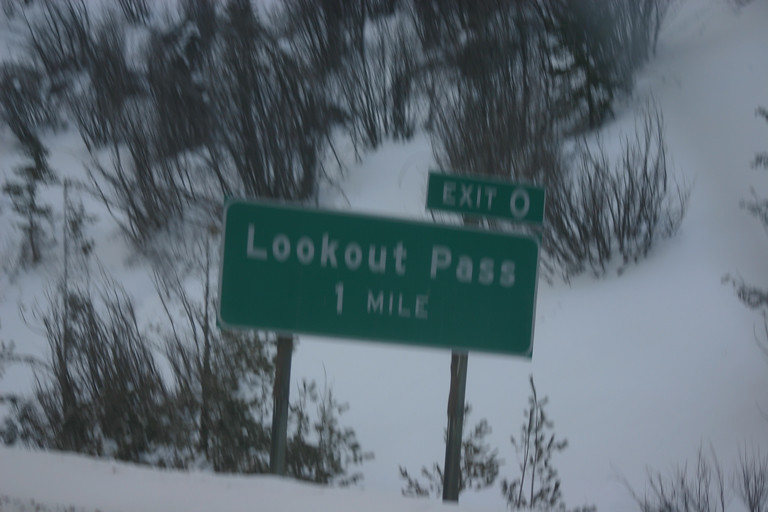This image, captured outdoors on a cloudy winter day, showcases a rural landscape dominated by a green road sign set against a snowy backdrop. The photograph is somewhat blurry but provides clear details of the highway sign, which is centered in the frame. The green sign, rectangular in shape with a white border and rounded corners, reads "look out past one mile." Above the upper right corner of this sign, a smaller additional green sign reads, "EXIT ZERO." All text is in lowercase except for "EXIT" and "MILE," which are in capital letters, with the numbers appearing in a digital format.

The sign is mounted on two wooden posts which partly disappear into the snow-covered ground. Surrounding the sign, the landscape is entirely blanketed in snow, with various vegetation standing out in sharp relief. The plants appear dead and weathered, ranging from smaller dried weeds to larger bare shrubs or saplings, all devoid of leaves typical of the harsh winter season. The terrain around the sign features a hill or mountain face in the background, while the sign itself seems to be positioned in a small gully or ditch along the road. The predominant colors in the scene are the stark white of the snow, the brown of the dead plants, and the green and white of the sign. There are no people or other objects visible in the photograph, emphasizing the isolation and stillness of the wintery landscape.